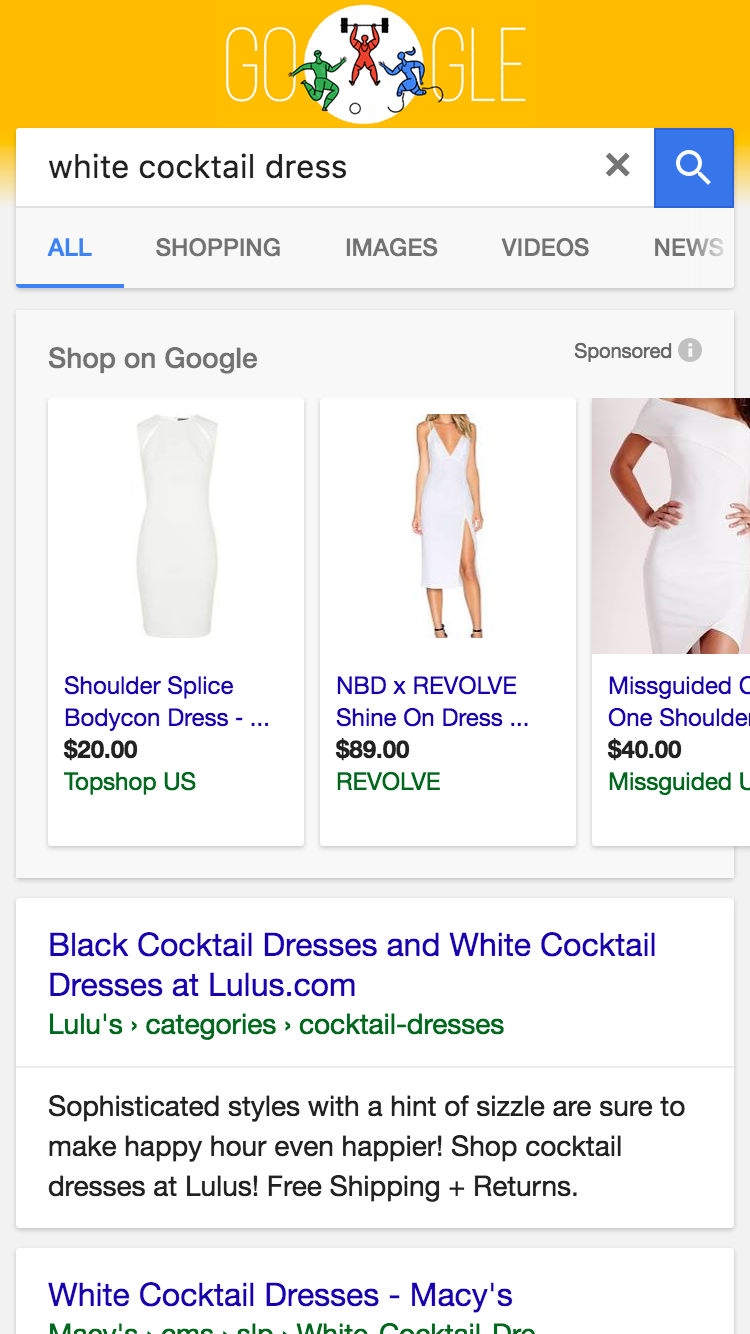The image is a screenshot of a Google search page captured on a mobile device, evident from its taller-than-wide orientation. The top of the page features a Google Doodle against a yellowish-orange background. The Google logo is stylized, with the second 'O' represented as a large white circle containing graphics of people exercising.

Beneath this logo is the search box, displaying the query "White Cocktail Dress." The "All" tab is highlighted, indicating the selected search category. Directly below, a sponsored section titled "Shop on Google" showcases three photos of dresses, complete with pricing and store information.

The first section of the search results includes an entry from lulus.com, listing categories leading to "cocktail dresses." The text snippet promotes sophisticated styles designed to make happy hour even happier, emphasizing free shipping and returns.

The second search result from Macy's is partially visible, showing the beginning of a listing for "White Cocktail Dresses" but is cut off at the bottom of the page.

Scrolling up reveals different tab options that were not selected: Shopping, Images, Videos, and News. The "Shop on Google" section displays images of dresses in a row. The first photo features a sleeveless dress, the second shows a model wearing a dress with a leg slit, and the third, partially cut off, depicts a model in a short white dress.